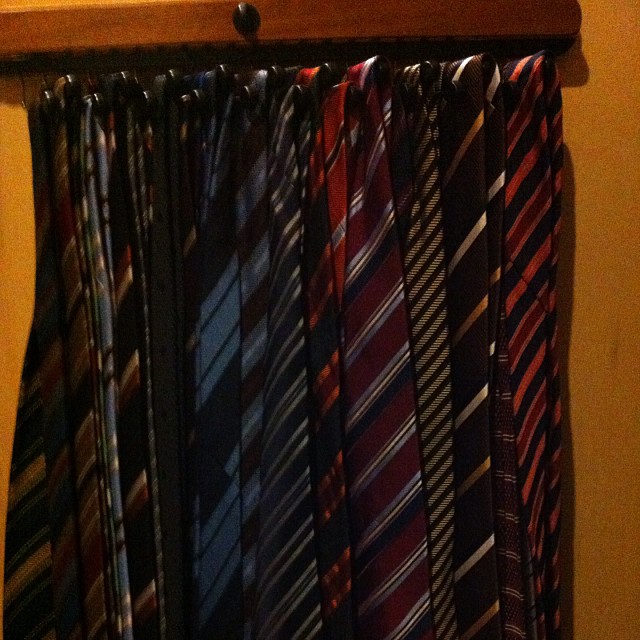This photograph showcases a tie rack mounted against a yellowish-orange wall, possibly within a wardrobe. The rack itself is constructed from wood, featuring a medium brown hue with a circular black knob-like piece in the center. Below this wooden bar, black metal or plastic hooks emerge, each bearing multiple ties. These ties, roughly thirty in total, predominantly feature diagonal stripes in a variety of color schemes including black, blue, red, brown, and shades in between. The stripes vary in width and pattern, adding to the visual interest. The lighting in the image is somewhat dim, creating shadows and a slightly vintage feel, reminiscent of the 1970s. The ties are meticulously arranged, draped from the top of the rack and cascading downwards, showcasing an orderly collection of business attire.